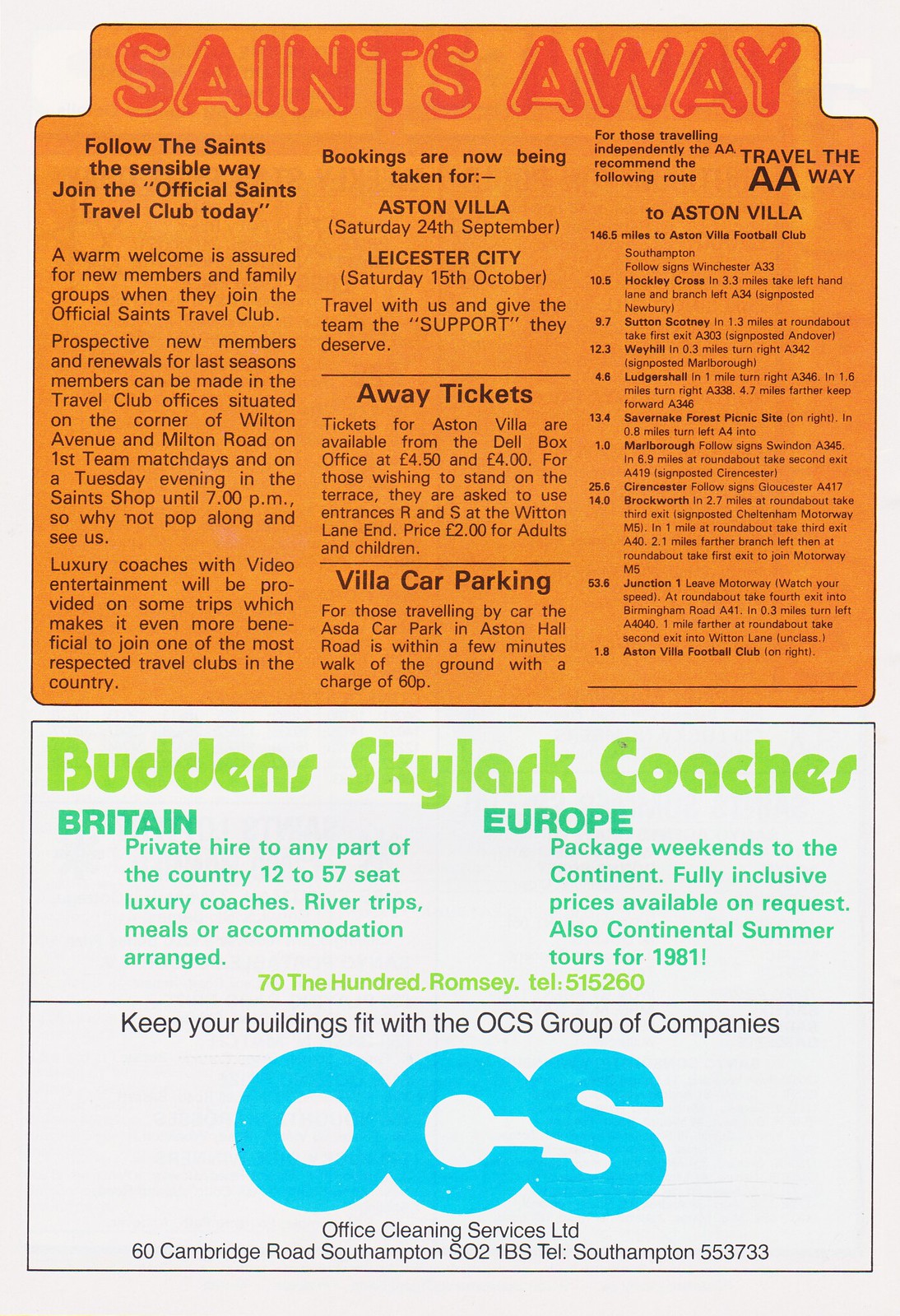This image is a scanned advertisement showcasing multiple services with a strong focus on the "Saints Away" travel club for sports enthusiasts. The top half of the advertisement has an orange background, headlined in prominent reddish text with "Saints Away." Just below, in smaller black text, it reads: "Follow the Saints the sensible way. Join the official Saints travel club today." The advertisement emphasizes a warm welcome for new members and family groups upon joining the club. 

Bookings for travel, including trips to Aston Villa and Leicester City, as well as services like away tickets and car parking arrangements, are prominently mentioned. Prospective members and renewals for last season's members can be handled at the travel club offices located at the corner of Wilton Avenue and Milton Road on first team match days, and until 7 p.m. at the Saints shop on Tuesday evenings. Additionally, luxury coaches with video entertainment are available for some trips, adding to the benefits of joining one of the most respected travel clubs in the country.

The bottom portion includes details for Bud and Skylark Coaches, offering travel packages within Britain and Europe. The very bottom of the advertisement features a logo and details for the OCS group, also known as Office Cleaning Services Limited, promoting their services with the tagline "Keep your buildings fit with the OCS group of companies," including their address in Southampton and contact information.